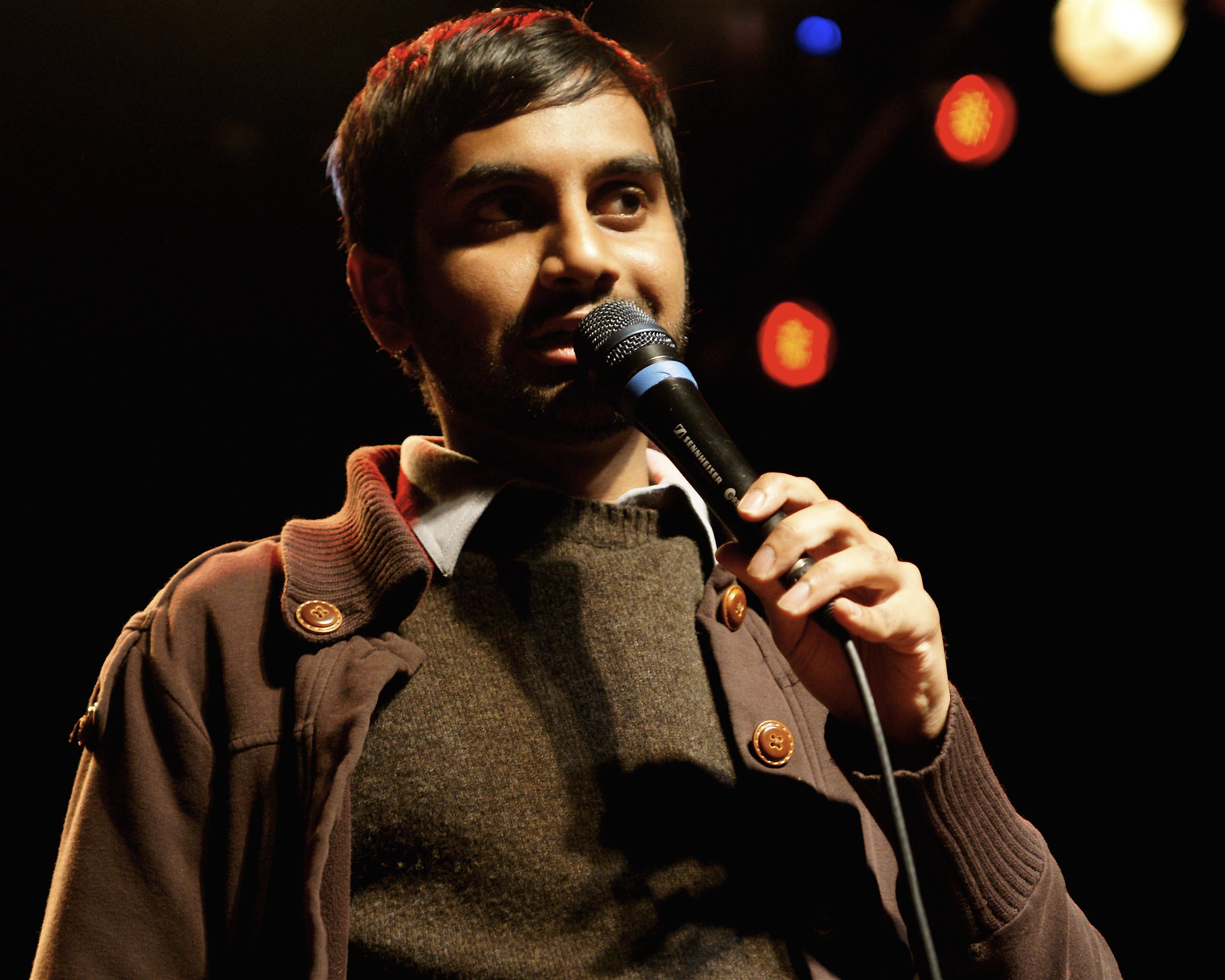This close-up photograph captures a man, who appears to be of Indian descent, holding a microphone to his mouth with his left hand. The man, standing slightly left of center in the dark background, is bathed in a spotlight that highlights his facial features. He has short, swept-over dark brown hair and is looking to the right of the camera with a slight smile on his face. He is dressed in a light brown jacket over a dark brown sweater, which in turn covers a white collared shirt. Above him to the upper right, there are several blurred lights in various colors—two red ones, a white one, and a blue one—adding depth to the otherwise black background. This setting, combined with his attire and the microphone, suggests he might be performing on a stage, possibly engaging in a singing or comedy act.